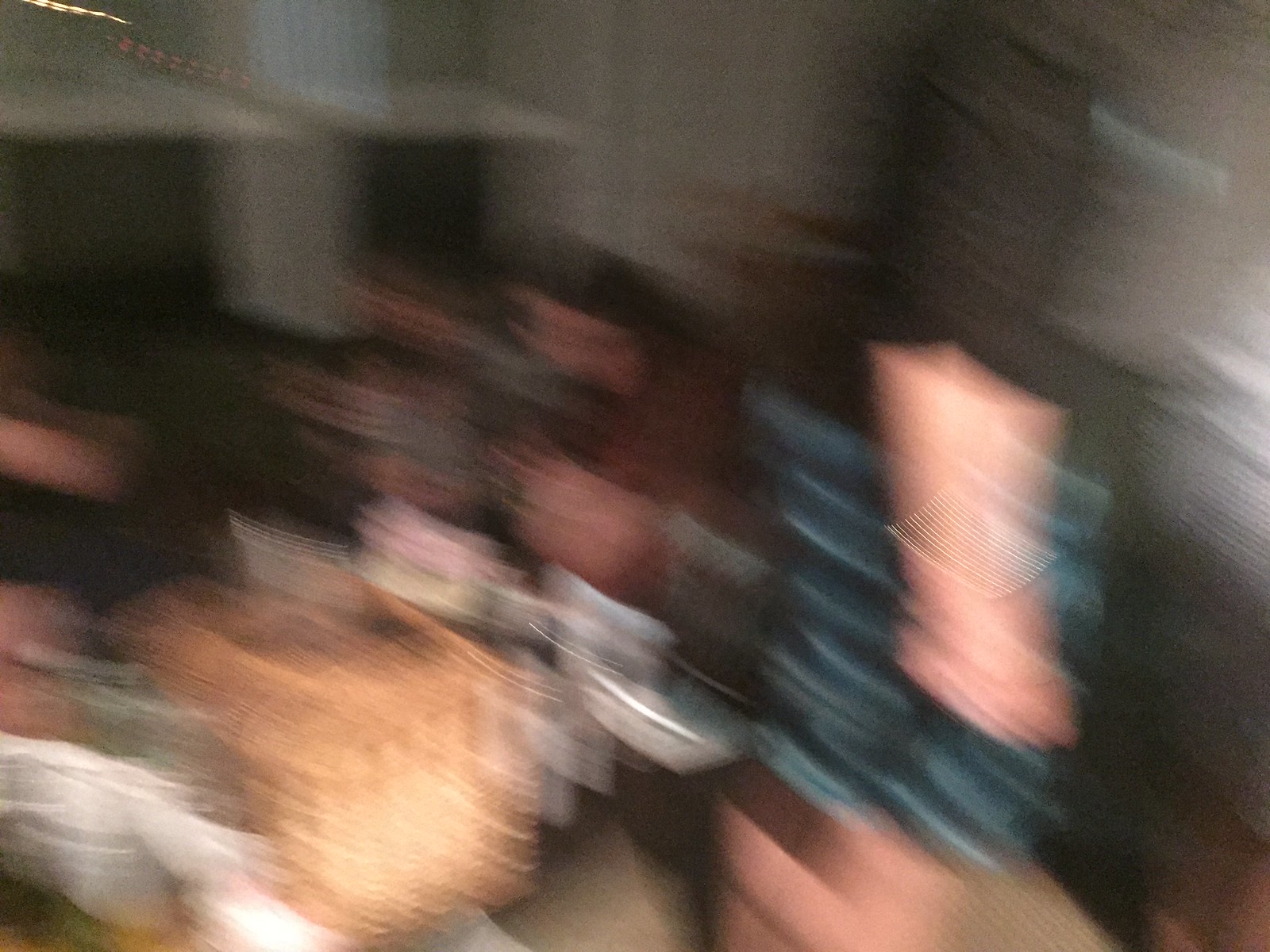A blurry image captures a person standing amidst a collection of round woven baskets and clay pots. The setting appears to be a room with interesting windowsills and a door visible in the background. Despite the movement and lack of clarity, the scene showcases a variety of colors including white, brown, light brown, and blue. A white wall serves as a backdrop, adding contrast to the earthy tones of the baskets and pots. Additionally, a vase can be seen, contributing to the eclectic assortment of items within the space.